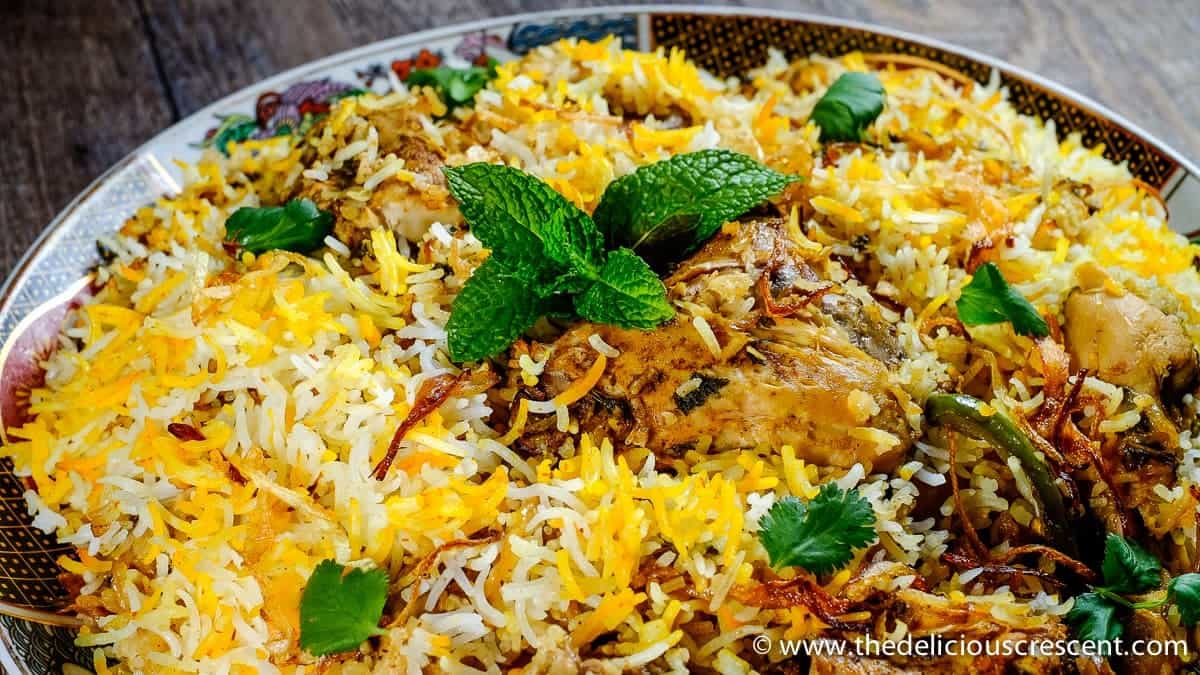This image features a beautifully presented food dish from www.thedeliciouscrescent.com. The dish is artfully arranged on an ornate plate with a gold trim and an intricate floral and diamond polka dot pattern, placed atop a wooden table. The centerpiece of the plate is a mix of white and yellow rice, generously seasoned and topped with well-cooked chicken pieces. The chicken, possibly baked, is garnished with fresh parsley or cilantro leaves, adding a touch of green to the vibrant array. Scattered among the rice and protein are slices of potatoes, and there are traces of red spices, possibly saffron or another exotic spice, enhancing the overall visual and flavor appeal. The dish includes additional herbs and possibly some peppers or onions, contributing to the aromatic and aesthetic elements of this delicious-looking meal.